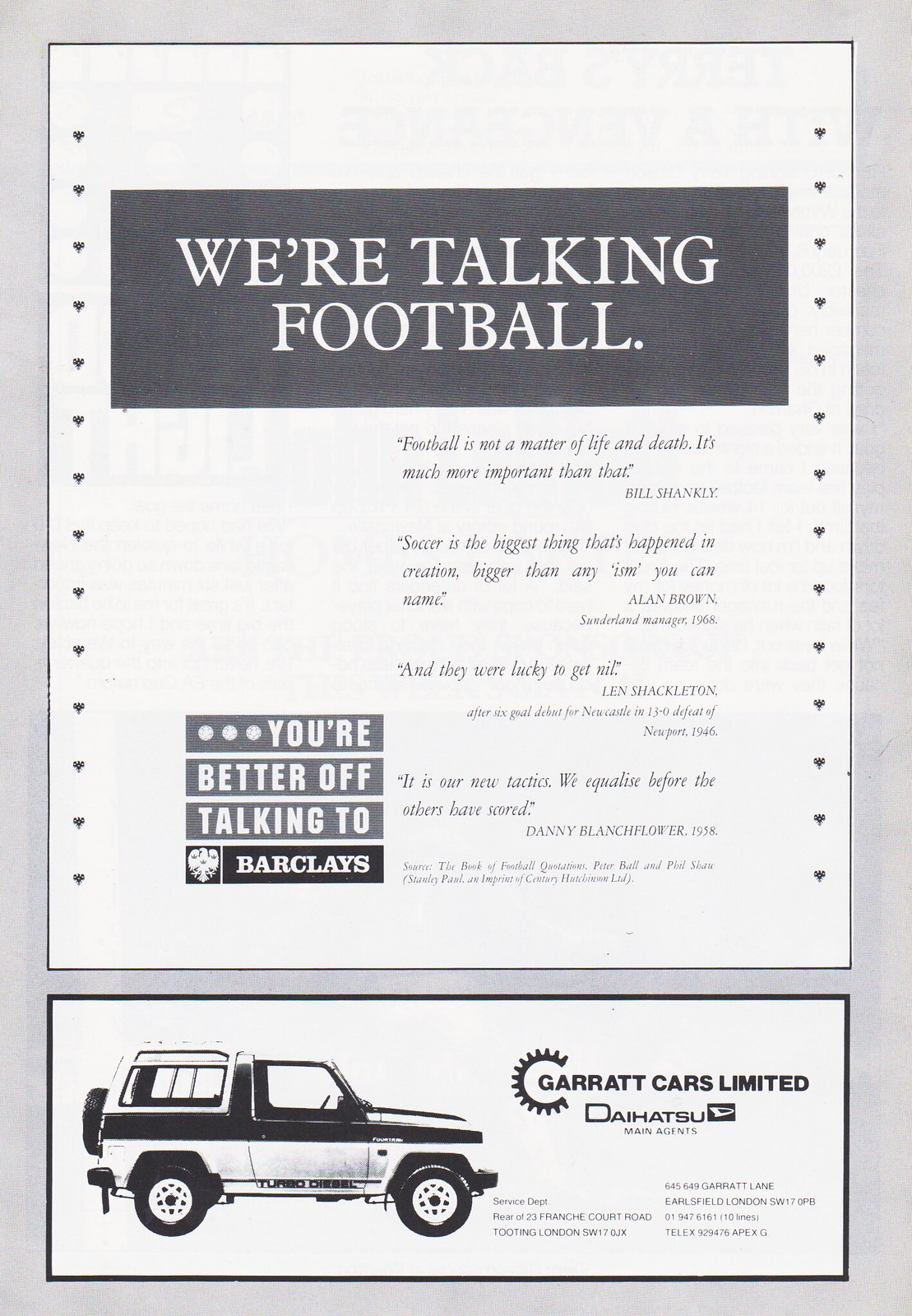This image features a football-themed flyer predominantly in black, gray, and white. The top half of the flyer, bordered by thin black lines, is dominated by a large, prominent gray block with the white text "We're Talking Football." Surrounding this text are two vertical rows of small, repeating symbols of the Barclays eagle, lining the left and right sides of the page. Below this heading are several quotations related to football: "Football is not a matter of life and death. It's much more important than that." — Bill Shankly, "Soccer is the biggest thing that's happened in creation. Bigger than any ism you can name." — Alan Brown, Sunderland manager, 1968, "They were lucky to get nil." — Len Shackleton, after his debut goal for Newcastle in a 13-0 defeat of Newport, 1946, and "It is our new tactics. We equalize before the others have scored." — Danny Blanchflower, 1958. Accompanying these quotes is a small text block that reads "You're better off talking to Barclays," set against a gray background. 

The bottom portion of the flyer contains an advertisement for Garrett Cars Limited, displaying a black-and-white image of a Daihatsu SUV. The text "Garrett Cars Limited" is prominently featured above the vehicle photo, followed by the word "Daihatsu." Below this are a few lines of small, hard-to-read text providing additional details about the dealership. The entire flyer is encased in a light gray border, complementing the overall monochromatic theme.